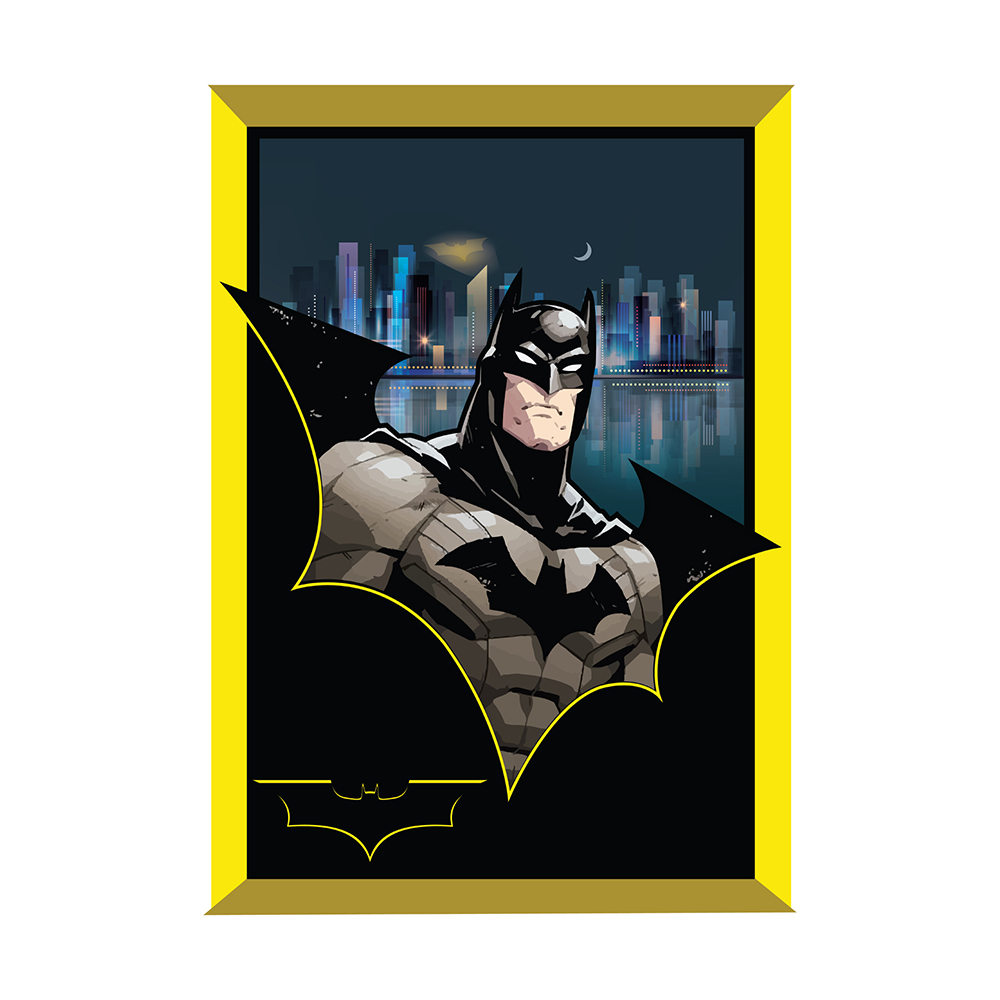This illustration depicts a striking image of Batman at its center, framed within a yellow, beveled border with brighter yellow on the sides and a darker yellow, almost brown on the top and bottom. Batman is shown in a powerful stance, facing slightly to the right while looking towards the viewer with his signature white eyes. He sports a tight gray, form-fitting suit, showcasing his muscular physique, and adorned with a black bat emblem on his chest. His iconic black cowl with pointed ears reveals only his mouth and square-shaped jaw.

Batman emerges from the silhouette of a larger, yellow-outlined bat logo at the bottom part of the frame, which stands out against a predominantly black background. The bat logo also appears in the bottom left corner, outlined in a subtle yellow pinstripe.

Behind Batman, a graphic design-style cityscape of Gotham unfolds, reflecting water and towering skyscrapers. Above this urban scene, a crescent moon hangs in a dark, dark blue or teal sky, punctuated by the illuminated Bat-Signal. The overall composition merges an illustration with elements of graphic design, presenting an evocative and visually compelling portrayal of the Dark Knight.